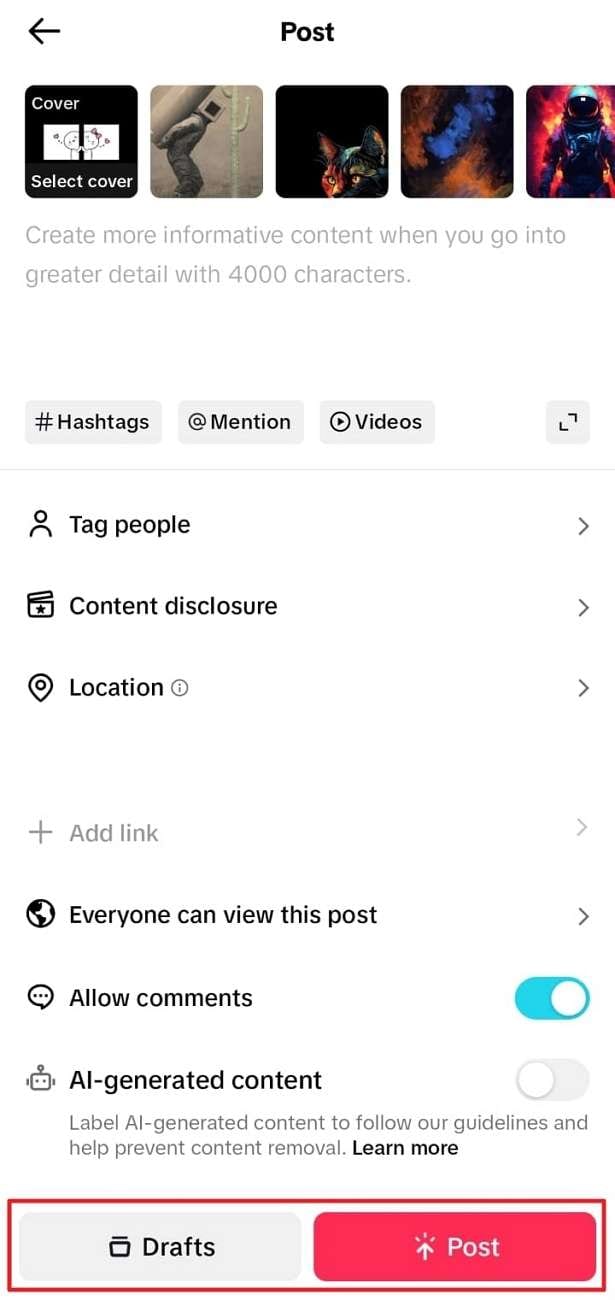Detailed Caption: 

This image is a mobile screenshot with a white background and black text. At the top left corner, there is a back arrow icon. The header prominently displays the word "Post." Below the header, there is a row of small album cover images, possibly thumbnails for some other content. 

Underneath this row, in light gray text, it reads, "Create more informative content when you go into greater detail with 4,000 characters." 

Below this instructional text, there are three gray buttons with black text: the first button reads "Hashtags," the second says "Mention," and the third is labeled "Videos."

Further down, there is a row of links that likely lead to drop-down menus; these links are labeled "Tag People," "Content Disclosure," and "Location." 

Following this is another section of light gray text that says, "Add Link." 

Underneath, three more actionable features are listed: "Everyone can view this post," "Allow comments" (this feature is turned on), and "AI generated content."

At the bottom of the screenshot, within a red rectangle, there are two buttons: one gray button labeled "Drafts" and another red button labeled "Post" with white text.